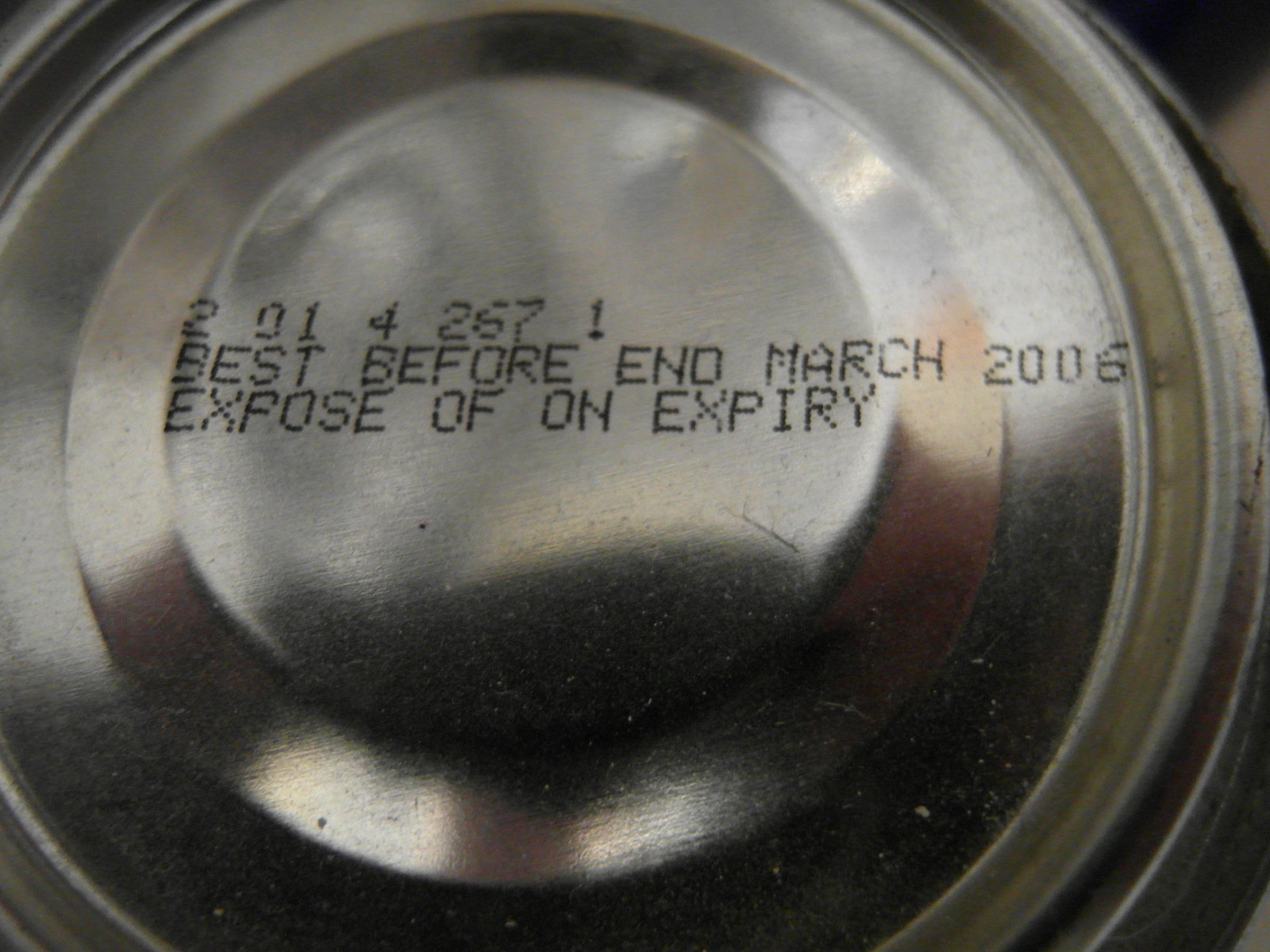This image is a close-up photograph of the bottom of a tin can, possibly containing food or soda. The can shows signs of aging and wear, with visible dents and indentations along its circular metal surface. The focal point of the image is the stamped text: "Best before end March 2006; dispose of on expiry." Additional markings include a series of numbers, "201 426 71." The photograph appears to capture the can in color, though the metallic nature of the object gives it a monochromatic look. Given today's date, the can is 18 years past its expiration, suggesting it is no longer safe for consumption and should be discarded.